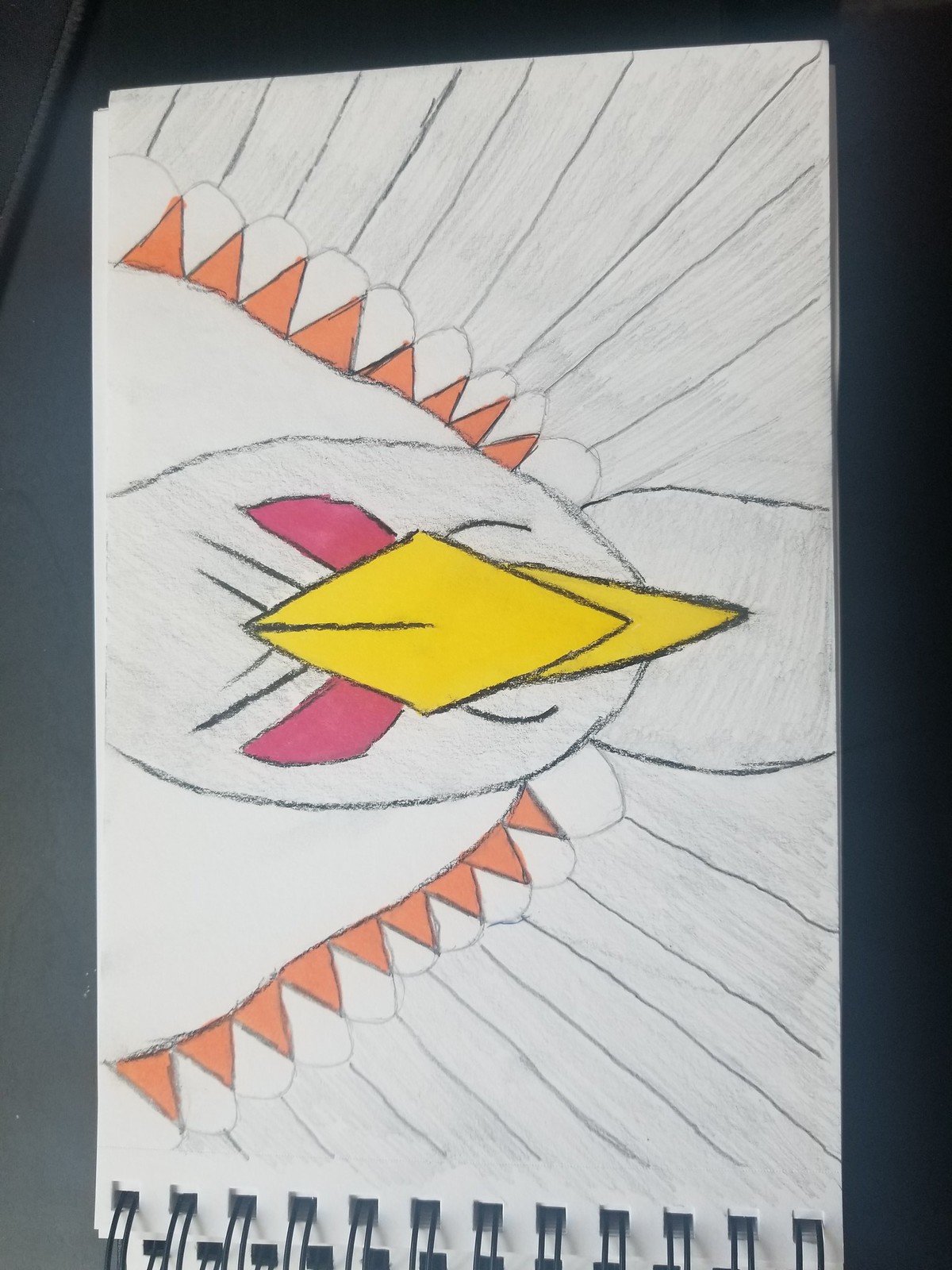This photograph captures a detailed drawing on a white piece of paper from a spiral sketchbook, which appears rotated on its side. The sketchbook has ring binding along the bottom. The drawing depicts an evil-looking bird with an oval head, featuring a triangular yellow beak and red, almond-shaped eyes. The eyes are slanted downward, giving it an angry expression, further emphasized by furrowed eyebrows. The bird is drawn in a predominantly black and white style, with some elements in color: the beak in yellow, the eyes in shades of purple to pink, and burnt orange triangular shapes along the upper edges of its unfurled wings. The background of the photograph is a navy-colored surface, adding contrast to the sketch. The overall style appears childlike and highly stylized.